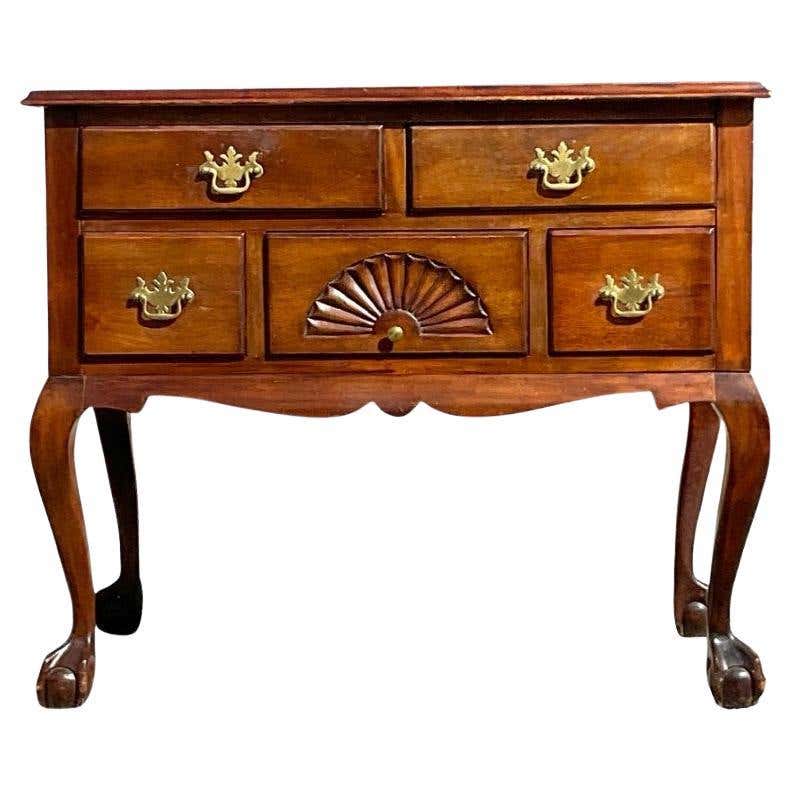The image depicts an antique-style wooden dresser set against a plain white background. This refined piece of furniture, likely mahogany, displays a light brown stain with a subtle reddish tint, and the finish is understated, not overly glossy. The dresser stands on four legs that feature an elegant claw-and-ball design. There are a total of five drawers: two square drawers at the top and three rectangular drawers beneath them. The drawers are adorned with intricate gold hardware, styled with a back plate that resembles an eagle with wings spread, enhancing the antique look. The central drawer at the bottom row is distinct, characterized by a small knob and a carved fan-like design. The piece is in excellent condition, free of nicks or marks, and the wood and brass elements are well-preserved, adding to the dresser's sophisticated charm. The detailed craftsmanship is particularly evident in the ornate carvings between the two front legs and the unique design on the center bottom drawer.